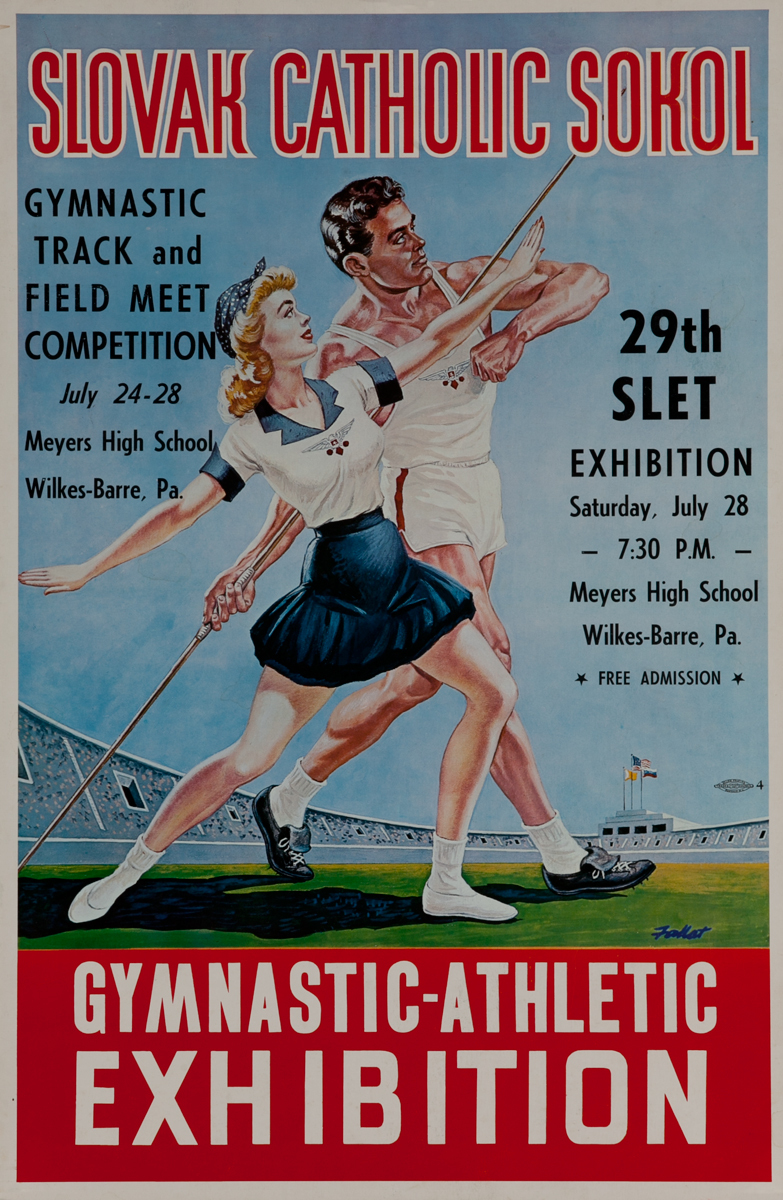The image is a vintage-style flyer for a sporting event, featuring a hand-painted illustration of a man and a woman on a grassy field with a stadium in the background. At the top, bold red text with a white border reads "Slovak Catholic Sokol," giving it a retro feel. The left side of the flyer announces a "Gymnastic Track and Field Competition, July 24th to 28th, Myers High School, Wilkes-Barre PA," while the right side promotes the "29th Slet Exhibition, Saturday, July 28th, 7:30 PM, Myers High School, Wilkes-Barre PA, Free Admission." The woman, in the foreground, is depicted with her left arm raised and right arm lowered, wearing a white short-sleeve shirt with blue accents, a blue pleated skirt, white shoes, and a blue handkerchief in her hair. The man behind her, dressed in a white muscle shirt and shorts with black cleats, appears poised to throw a javelin. At the bottom of the flyer, white letters on a red banner read "Gymnastic Athletic Exhibition."